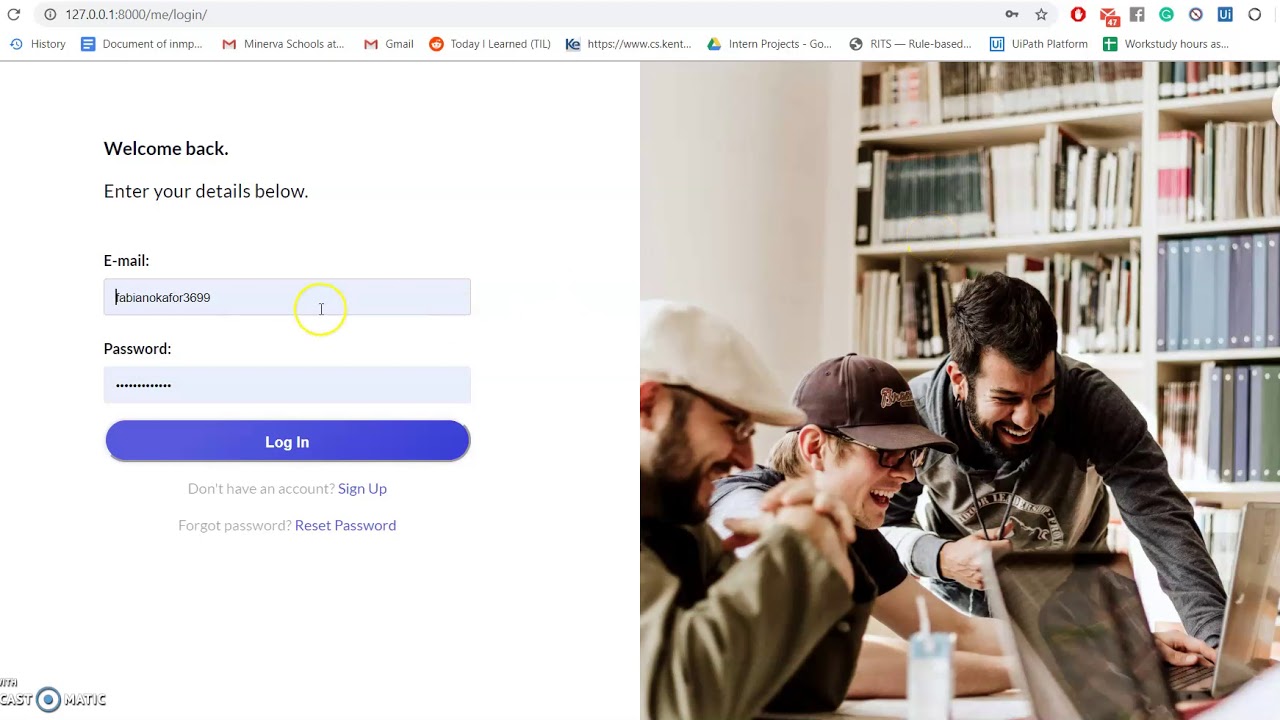This is a detailed screenshot of a web browser on a desktop or laptop computer displaying a locally hosted website at the address 127.0.0.1. The website appears to be under development, only available on the user's local machine or network. The image is in a landscape widescreen format.

On the left side of the screenshot, there's a clean white field with black text that reads: "Welcome back, enter your details below." Directly below this text is an input box labeled "Email," which has been filled in with "Fibonacci43699." Below the email input is a password field, with the entered password obscured by a series of asterisks for privacy. Positioned beneath the password field is a prominent purple "Login" button.

Further down, the text prompts the user with additional options: "Don't have an account? Sign up" (with "Sign up" being a clickable hyperlink) and "Forgot password? Reset password?" (with "Reset password?" also a clickable hyperlink).

On the right side of the screenshot, an engaging image features three people sitting in front of a laptop, looking at the screen with smiles and laughter, suggesting collaboration or shared enjoyment.

At the bottom of the image, there's a watermark that reads "CastMatic," with a distinctive blue bullseye logo placed between "Cast" and "Matic."